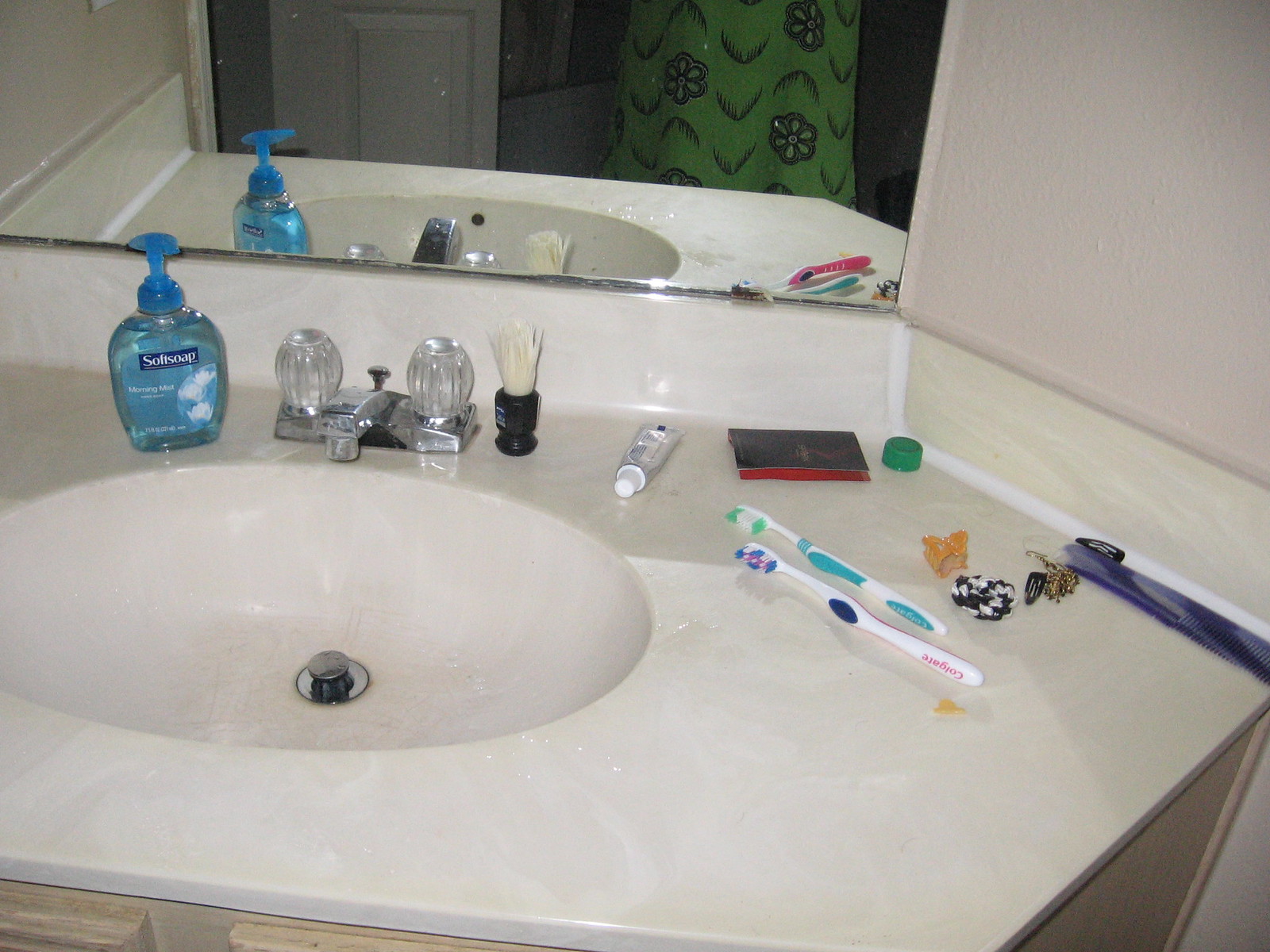The close-up photograph captures the detailed clutter of a bathroom countertop, which is finished in a subtle off-white marble. The frame shows portions of light brown wooden cabinetry at the bottom corners. The sink, slightly stained with yellowing around the drain, features a small, chrome faucet with distinctive, dated 1980s-style clear knobs, which are more cylindrical than spherical. To the left of the faucet, a blue bottle of Softsoap with a "Morning Mist" label stands in front of the mirror. On the right, a shaving brush with its bristles pointing upward is balanced on the handle. Scattered around the sink area are additional personal items, including a white toothpaste tube, two toothbrushes lying flat, and several small hair clips. The mirror above the sink reflects a green shower curtain adorned with floral patterns and bird-like shapes, providing a glimpse into the room's overall modest, vintage aesthetic.